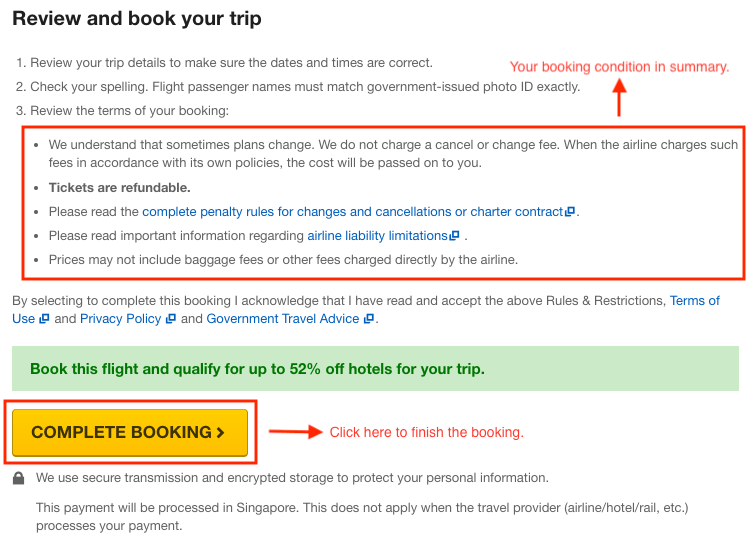**Descriptive Caption for the Image:**

The image showcases a detailed booking page for a flight. At the top, users are prompted to review and book their trip, ensuring all details such as dates and times are accurate. The summary of booking conditions highlights that while the platform does not charge fees for changes or cancellations, any fees imposed by the airline will be passed on to the customer. It mentions that tickets are refundable and advises users to read the complete penalty rules for changes, cancellations, and charter contracts. Important information regarding airline liability limitations is also provided.

Additionally, the text notes that baggage fees and other charges by the airline may not be included. To proceed with the booking, users must acknowledge that they have read and accept the rules and restrictions, terms of use, privacy policy, and governmental travel advice. The page encourages booking by offering up to 52% off on hotel reservations once the flight is booked. Finally, it assures customers that their personal information is protected through secure transmission and encrypted storage, and it specifies that the payment will be processed in Singapore unless handled directly by the travel provider, airline, hotel, or rail service.